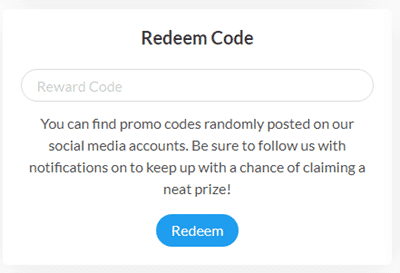This is a screenshot of the interface where users can enter a promo code. The primary element is a light gray box with a matching border, set against a white background. At the top center of the box, the heading "Redeem Code" is displayed in a dark gray or black font. Below this heading is an empty text field labeled "Reward Code." Beneath the text field, a passage reads: "You can find promo codes randomly posted on our social media accounts. Be sure to follow us with notifications on to keep up with the chance of claiming a neat prize." At the bottom of the box is a pill-shaped, light blue button with the word "Redeem" in a white font.